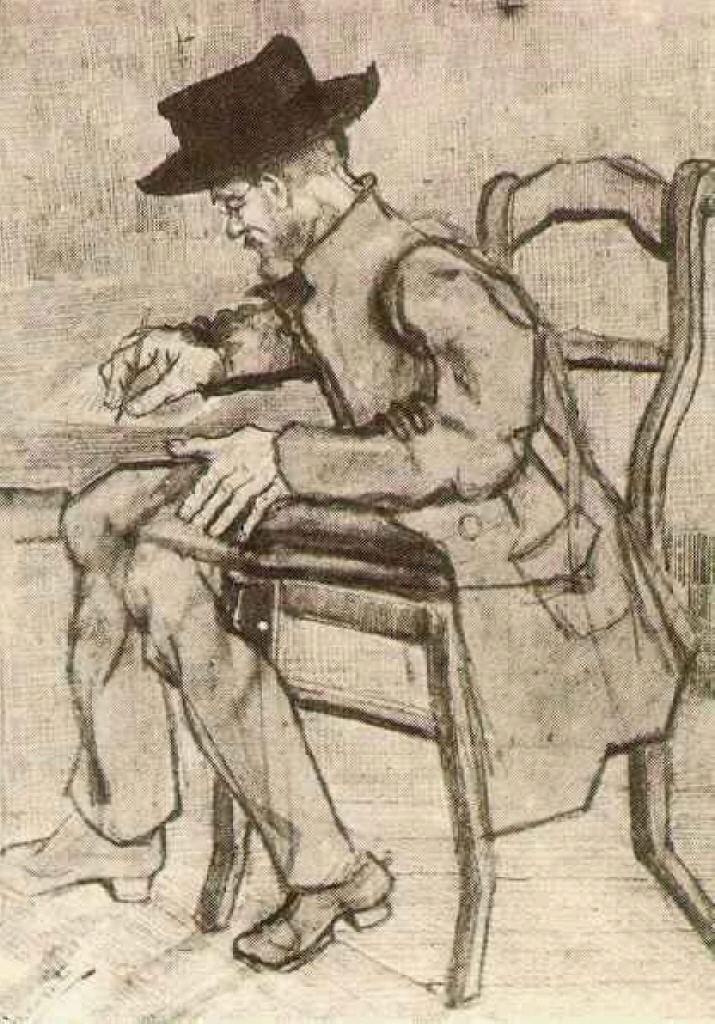The image is a detailed sketch, possibly using shades of charcoal, of a man seated in a wooden, armless chair with a ladder-back design. He is dressed in a long coat or cloak that drapes over the chair, and pants paired with pointy dress shoes. The man wears a stylized black or dark gray hat and glasses, and his scale appears slightly altered, particularly noticeable in his over-large hands. He is depicted in a three-quarters view from the front and left side, leaning forward and writing or drawing in a book or on a page with his right hand, while his left hand rests on his crossed leg. The sketch employs cross hatching for shading, and the background consists of varying lines in charcoal, with possible hints of brown and white. The overall scene appears monochromatic, focusing entirely on the solitary figure and his concentrated activity.